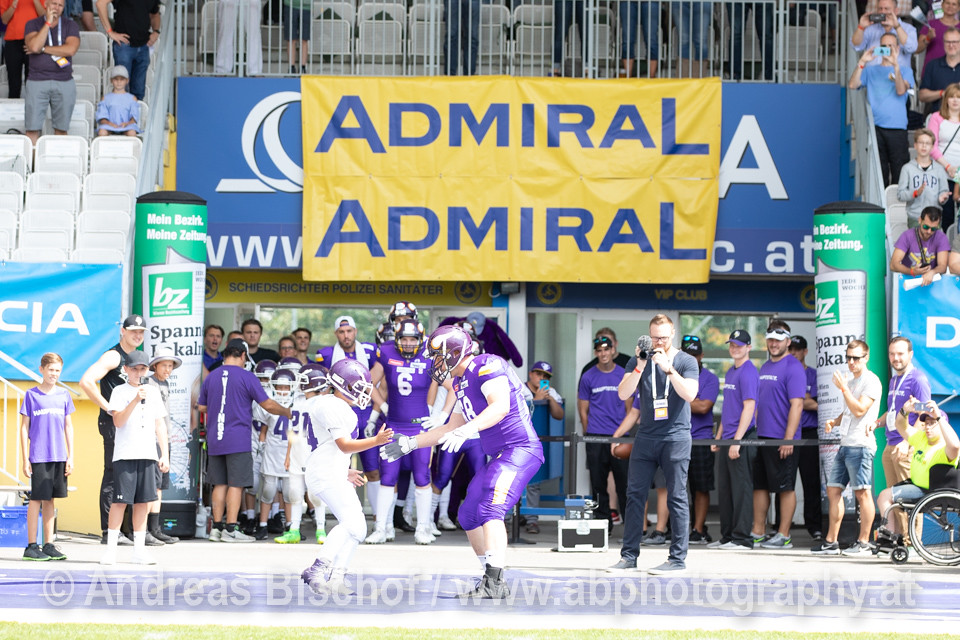In this vibrant and detailed image taken by Andreas Bischoff (www.abphotography.at), a thrilling scene unfolds at a stadium during the daytime, under the clear blue sky. At the heart of the photograph, prominently placed in the center, a heartfelt moment captures a young boy in a white football uniform with a purple helmet and number, high-fiving an adult football player donned in a purple uniform with gold accents and a yellow helmet. This interaction between the youth and the professional player forms the focal point of the image, evoking a sense of inspiration and connection across generations of the sport.

Surrounding this central scene, several other football players in purple jerseys and pants with gold helmets can be seen, either appearing from a tunnel entrance or mingling on the field. To the left of the frame, young kids dressed in casual shorts and t-shirts watch in awe, adding to the lively atmosphere. On the right, spectators, possibly trainers or managers, stand clad in purple t-shirts while a photographer with a camera and lanyard captures the unfolding moments.

Above this dynamic gathering, a yellow banner with bold blue letters reading "Admiral Admiral" hangs over a tunnel entrance, hinting at German origins with additional German signage on the pillars. Beyond this entrance, white stadium seats filled with fans extend into the upper corners of the image, completing the scene with their excited presence.

Colors are visually rich and varied, with dominant hues of purple, gold, white, and yellow interspersed with touches of blue, lime green, gray, and black, adding to the vibrant tapestry of this evocative sports moment. The detailed composition and the interplay of different elements underline the energy and excitement of the event, encapsulating a perfect snapshot of a spirited football match day.